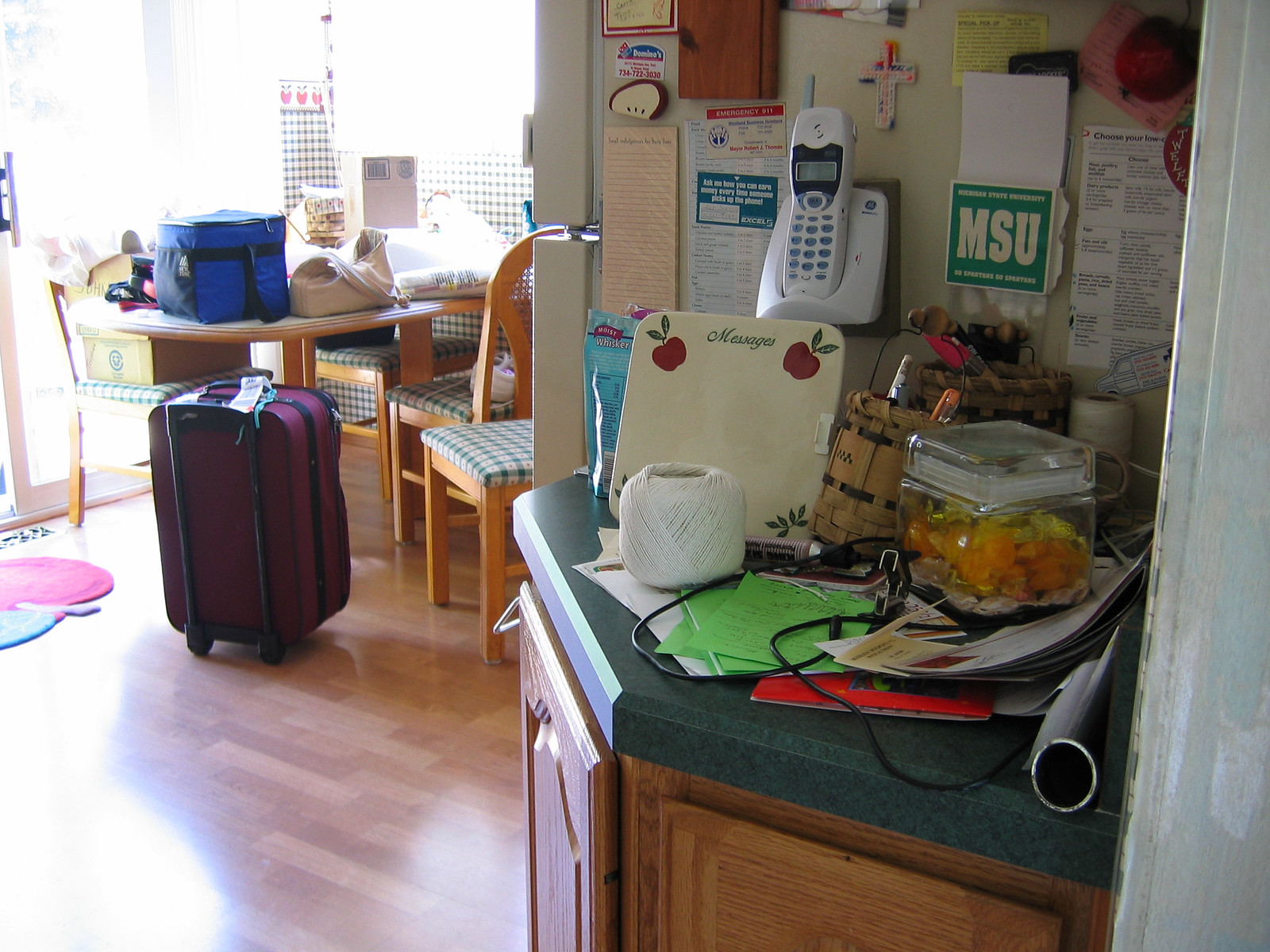The image depicts an extremely cluttered and disorganized kitchen. To the left, there is a small area by the telephone mounted on the wall, which seems designed to function as a desk for notes and miscellaneous items, now piled with various objects. Among the clutter, a ball of string is tangled and a board for writing notes is missing its pen. A square glass jar filled with butterscotch candies sits prominently. An unidentifiable gray roll and a haphazardly thrown cord add to the disarray.

The wall is densely cluttered with items such as a cross, an MSU sign, and numerous scattered notepads. The kitchen table is equally chaotic, covered with an assortment of items including a cooler, a pocketbook, and a box containing unknown contents. The chairs around the table are not positioned neatly; one holds a box, and others are pulled back irregularly. 

A purple luggage bag with an airline tag further adds to the confusion, accompanied by what might be a booth located behind the table, although it’s difficult to ascertain due to the sheer amount of clutter. Various bags are scattered around, contributing to the mess. A sliding door in the background lets in daylight. On the floor, a pink mat with blue details lies near a vent, probably for air conditioning.